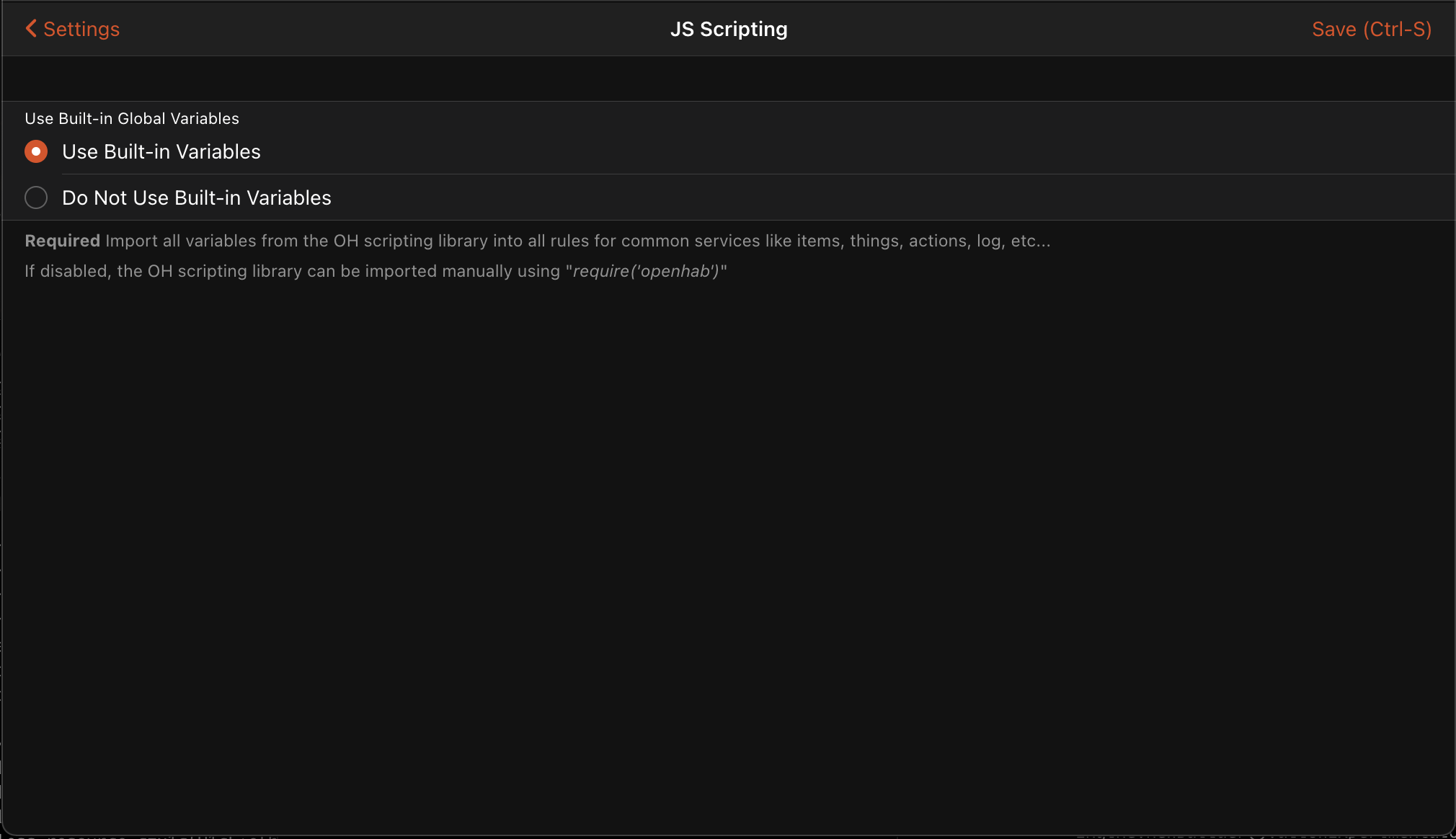**Detailed Caption:**

At the top of the image, there is a dark gray header. Towards the left side of this header, the word **"Settings"** is displayed in a red font, accompanied by a left-pointing arrowhead. Centrally positioned within the header is the text **"JS Scripting,"** written in bold white font, where "J" and "S" are capitalized. To the right, in the same red font, it says **"Save (CTRL-S)."**

Beneath the header, the background transitions to black. There is a rectangular section featuring the same dark gray background as the header. In this section, the phrase **"Use built-in global variables"** is written in small white text.

Below this phrase are two tick options:

1. The first option states **"Use built-in variables."** This option is selected, indicated by a red-bordered circle with a white dot in the center to the right of the text.
2. The second option reads **"Do not use built-in variables."** This option is represented by a light gray circle outline.

Each option is separated by a thin, light gray line divider. At the bottom of this section, **"Required"** is written in bold gray lettering. Following this, in non-bold font, the description continues: **"Import all variables from the OH Scripting Library into all rules for common services like items, things, actions, log, etc..."** The description also states: **"If disabled, the OH Scripting Library can be imported manually using "*require('openhab');*"** with the citation in italicized quotations.